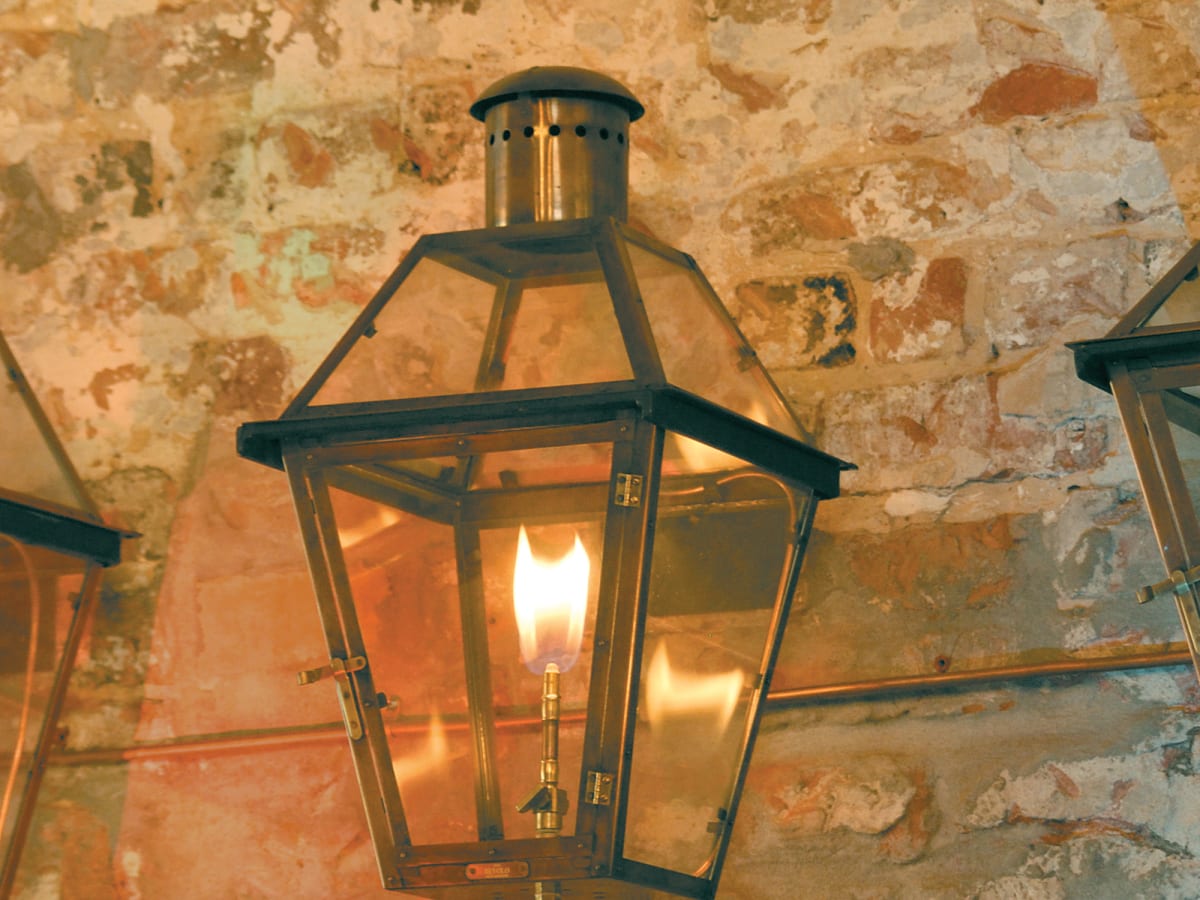The image features a rectangular, worn brick wall with a cream-colored background interspersed with reddish-copper and blackish spots, adding to its rustic and old-fashioned charm. Dominating the center of the composition is a metal lantern with clear glass panels, in which a flame is visibly flickering, evoking the appearance of an old-fashioned oil lamp. The lantern appears relatively new in contrast to the aged wall, giving it a decorative appeal. On both the left and right edges of the image, the very edges of two more similarly styled lanterns can be seen, partially cut off. The overall scene is bathed in an amber glow, likely from the lantern's light, imparting a warm and nostalgic ambiance to the photograph.